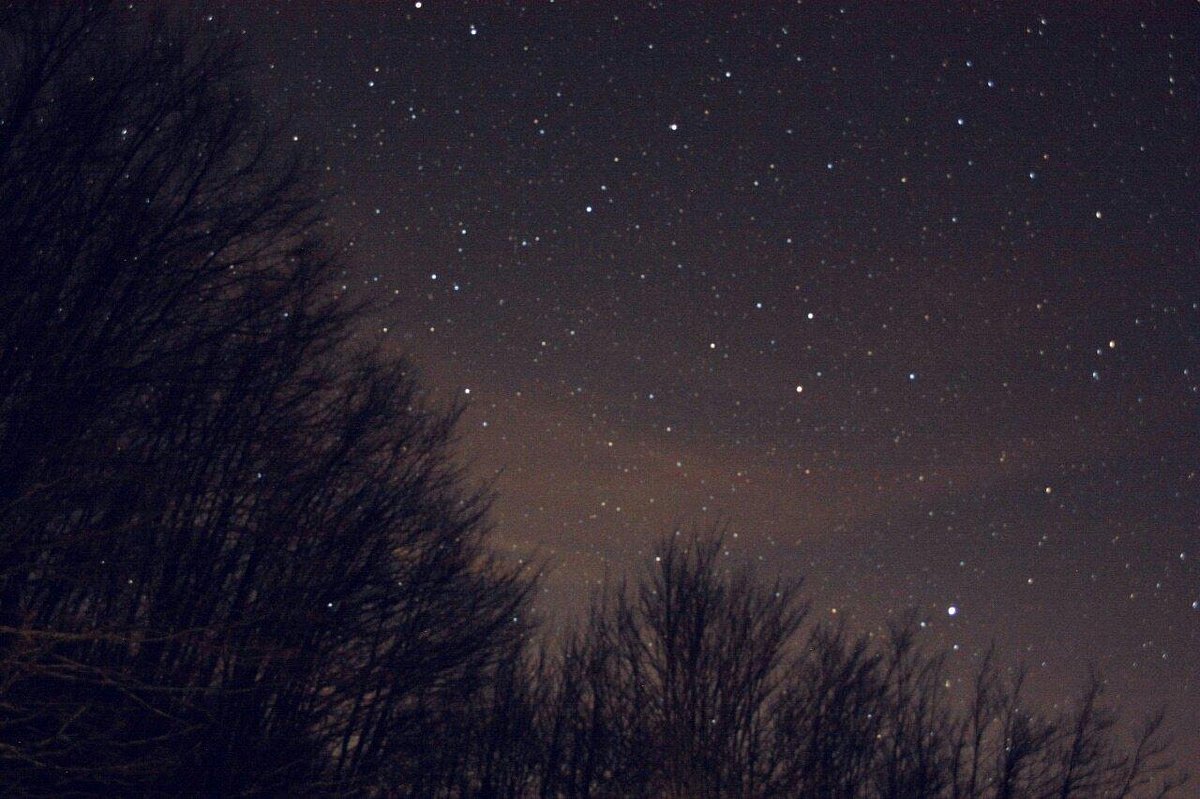In this captivating nighttime photograph, we witness an incredibly starry sky, unobscured by light pollution, suggesting it's taken far from city lights, possibly in a forest setting. The sky is a deep, dark canvas, particularly in the upper right corner, showcasing a dazzling array of stars, possibly the most you could ever see in one night. As your eyes travel downward towards the center, the sky brightens up with an amberish hue, potentially hinting at moonlight or a faint suggestion of northern lights, adding a mystical quality to the scene. Dominating the left side, extending from the top left to the bottom right, are trees that appear barren, likely indicating winter or late autumn. These trees, dark and leafless, frame the bottom of the image, adding depth and contrasting the luminescent sky. The overall palette of the image is a mesmerizing blend of black, bluish-gray, and hints of orange-red undertones, painting a serene and enchanting picture of nature's nighttime splendor.